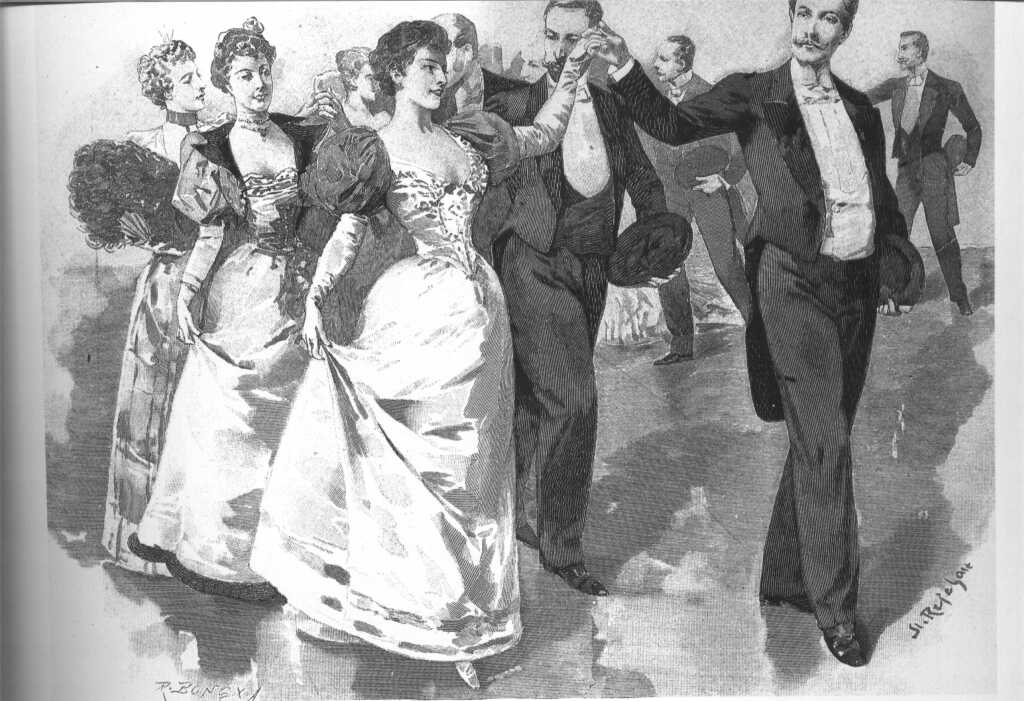In this black-and-white, pencil-drawn illustration from the 1850s, groups of men and women are depicted walking in lines that curve to the right. The women, positioned on the left, wear long, white ball gowns with puffy sleeves, tight bodices, and long gloves extending past their elbows. Their hair is elegantly pinned up. The men, to the right of the women, are dressed in black tuxedos with white dress shirts and bow ties. Some men also wear black vests and sport handlebar mustaches, with the man in the foreground showcasing a curved mustache. Each man carries a hat in his left hand while holding the hand of his female partner with his right. The scene appears to be a formal dance, with about six or seven couples participating in this traditional Victorian setting. The word "J. Refayar," presumably the artist's signature, is visible in the bottom right corner.